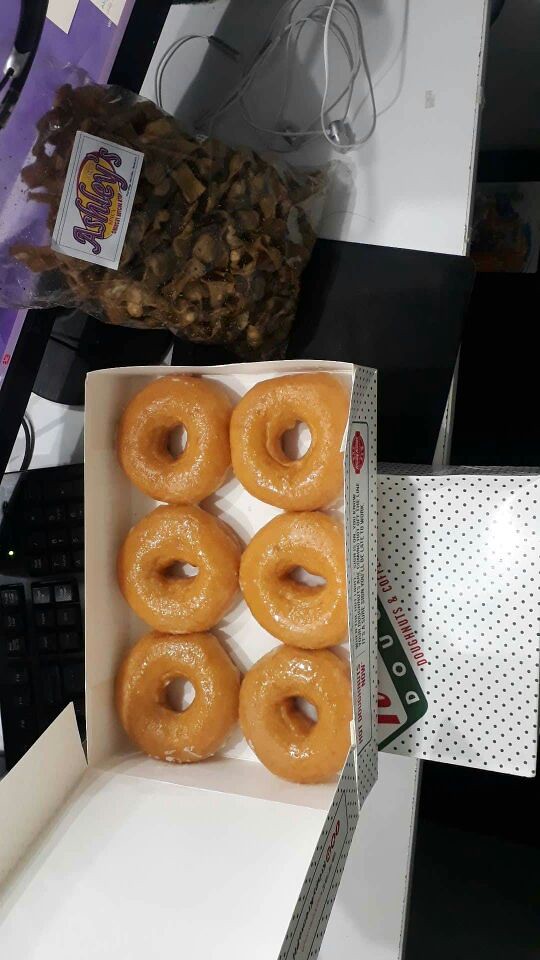In the image, a top-down view reveals a partly open Krispy Kreme doughnut box in the bottom left corner, containing six glazed doughnuts with a glossy sheen. The white box with a black dotted pattern sits atop a closed Krispy Kreme box, also white with black dots and red font reading "Donuts and Coffee." Positioned just above the doughnut boxes, there is a bag labeled "Ashley's" in purple, possibly containing brownish snack mix or dog treats. The scene is set against black and white tile flooring, with the doughnut boxes located next to a black keyboard, noticeable on the left side of the image. Additionally, a laptop and a monitor are seen in the top left corner, along with a visible cable behind the bag of "Ashley's" snacks.